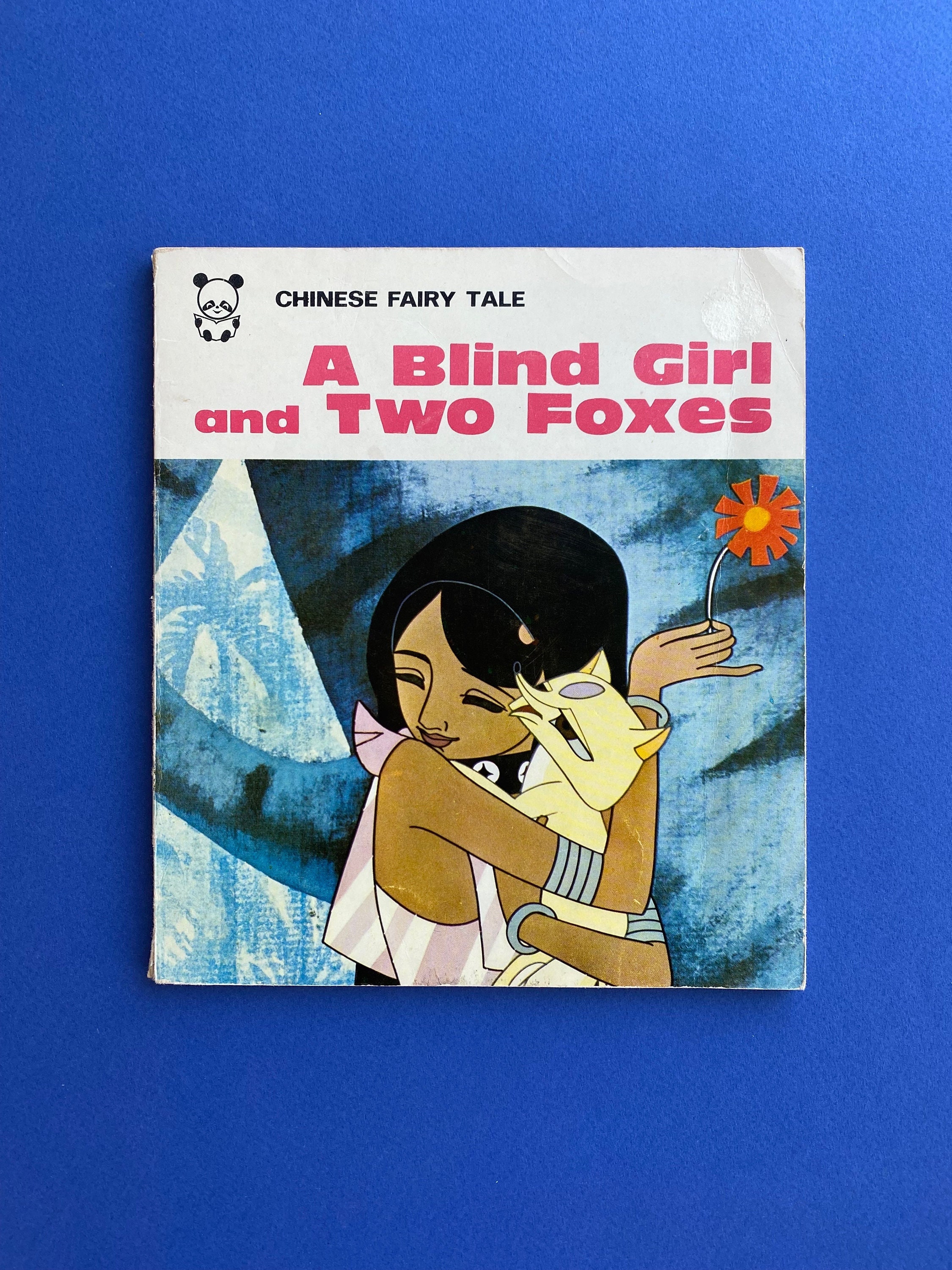The cover of this small, square children's book features a vivid illustration central to the theme of a Chinese fairy tale. In the top left corner, a small panda bear is depicted next to the text "Chinese Fairy Tale" written in black. The prominent title "A Blind Girl and Two Foxes" appears in bold, red lettering. The book cover, though slightly bent at the right edge with the spine showing a bit of wear at the bottom left, draws much of its charm from the illustrated scene below the title.

The image showcases a young girl with dark hair and skin, warmly smiling with her eyes closed as she hugs a pale tan fox with a distinctive gray spot between its eyes. The girl, dressed in a pink and white sleeveless dress adorned with shoulder ties, wears armbands and holds a vibrant red flower with a yellow center in her right hand. The background, a deep blue, features delicate palm trees, enhancing the ethereal and dreamlike quality of the illustration. The book itself lays upon a royal blue background, further accentuating the fairy tale's nocturnal and magical atmosphere.